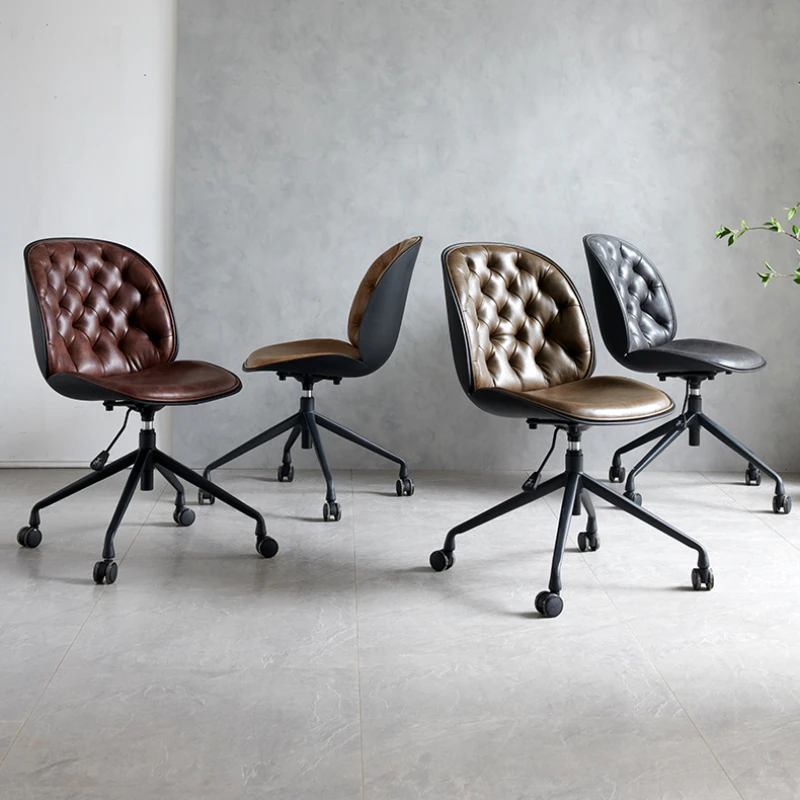The photograph depicts a minimalist office setting with a gray background wall and a floor made of gray or white stone tiles. Positioned in a row from left to right are four tufted office chairs on rolling casters, each equipped with height adjusters. The chair on the left features a dark brown leather seat with tufted buttons, a black backrest, and black legs. The next two chairs are identical, showcasing bronze-colored tufted leather seats, also with black backs and legs. The chair on the far right is upholstered in smoke-gray tufted leather and similarly has a black back and legs. All the chairs are armless and feature a uniform black plastic back support, lending a cohesive aesthetic to the scene. The room appears to be well-lit by natural light coming from a window on the right, with a hint of greenery just visible at the extreme right edge of the image.